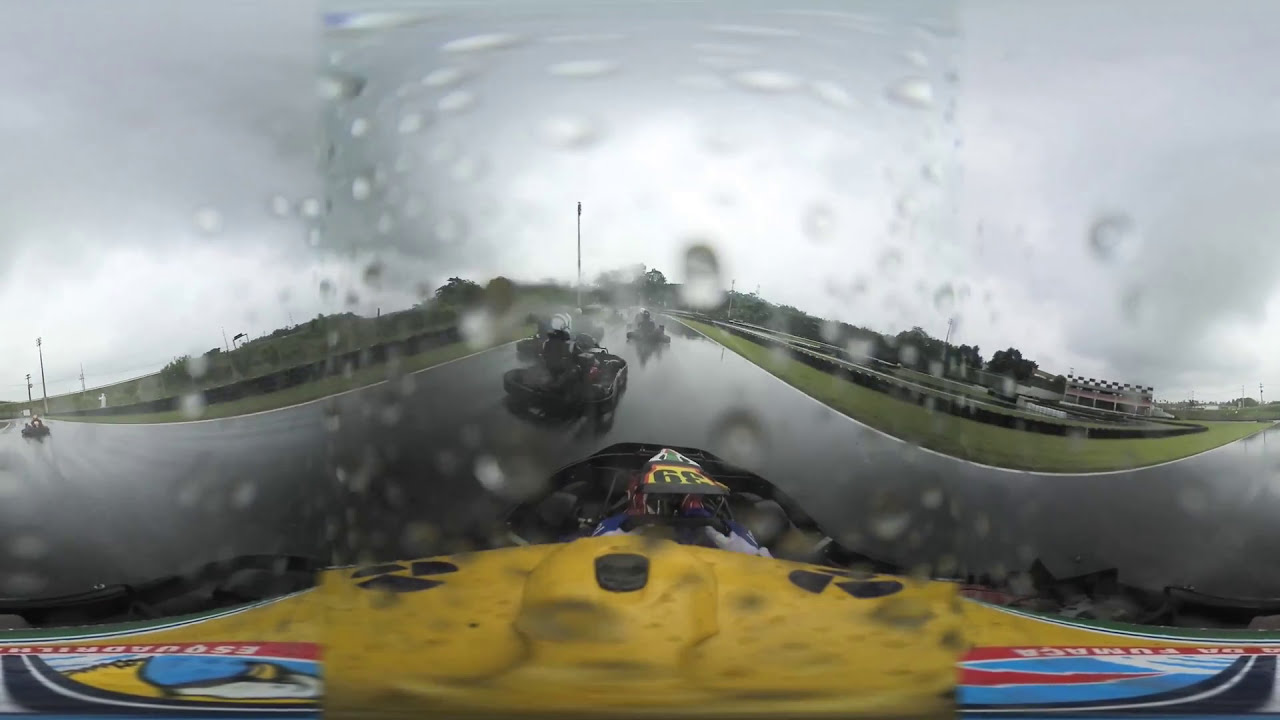The photo is a detailed 360-degree view from inside a race car on a racetrack during a rainy day. Through the windshield, raindrops are visible, and the sky is dark and cloudy. The car's hood, prominently yellow, features red and blue designs, along with a radioactive sign on both sides. There's a partial race number, likely 39, displayed on it. Stickers with a red outline, blue centers, and white and yellow elements are also spotted at the bottom corners of the hood. Several stripped-down race cars are seen ahead, with one approaching from the rearview. The track appears to be a circular layout, with fencing and safety barriers or tires along the sides of the road to mitigate crash impacts. The overall scene captures the tense atmosphere of a race under challenging weather conditions.